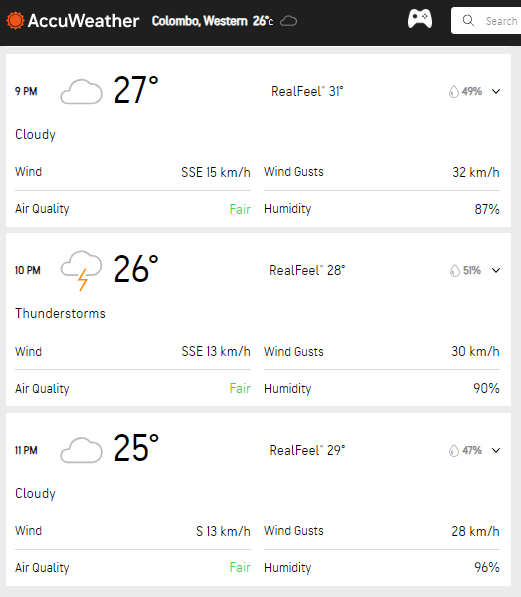The image depicts a weather forecast page with a white background. At the top, it features the heading "AccuWeather," followed by location and temperature details: "Colombo, Western, 26°C." 

The page includes a sidebar with icons representing a gaming pad, controller, and magnifying glass with the text "search" next to it. The primary forecast details are as follows:

For 9 PM, it shows:
- Icon: Cloud
- Temperature: 27°C
- "Feels Like": 31°C
- Indicator: Raindrop with "49%" and a downward arrow
- Condition: Cloudy
- Wind: SSE at 15 kilometers per hour
- Wind Gusts: 32 kilometers per hour
- Air Quality: Fair
- Humidity: 87%

For 10 PM, it displays:
- Icon: Cloud with a zigzag (lightning symbol)
- Temperature: 26°C
- "Feels Like": 28°C
- Indicator: Raindrop with "51%" and a downward arrow
- Condition: Thunderstorms
- Wind: SSE at 13 kilometers per hour
- Wind Gusts: 30 kilometers per hour
- Air Quality: Fair
- Humidity: 90%

For 11 PM, it presents:
- Icon: Cloud
- Temperature: 25°C
- "Feels Like": 29°C
- Indicator: Raindrop with "47%" and a downward arrow
- Condition: Cloudy
- Wind: SSE at 13 kilometers per hour
- Wind Gusts: 28 kilometers per hour
- Air Quality: Fair
- Humidity: 96%

The layout efficiently conveys the upcoming weather conditions, including temperatures, precipitation chances, wind speed, and additional atmospheric details.